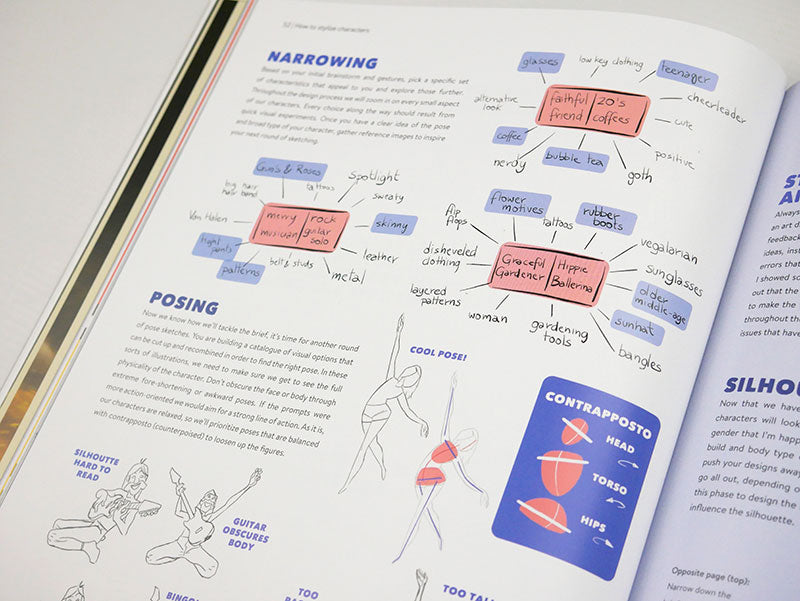This image captures a detailed view of an open textbook on a white or light gray table, positioned at a right-hand diagonal. The textbook page features a clean white background with various sections and diagrams designed to teach drawing techniques and character design.

In the upper left corner of the page, bold blue text reads "Narrowing," followed by a detailed paragraph in black print that is too small to read. Beneath this, a red rectangle contains highlighted words in blue, surrounded by lines pointing to terms like "Mary," "rock guitar solo," "skinny," "spotlight," and "guns and roses."

Further down, another bold blue title "Posing" introduces a paragraph explaining various posing techniques. Below this, in blueprint, annotated diagrams of people with guitars illustrate different poses, with terms like "silhouette," "guitar obscure body," and additional outlines detailing head, torso, and hip positions.

On the right side of the page, two red rectangles present a descriptive flow chart with terms like "faithful friend," "20s copies," "teenager," "glasses," "coffee," and "bubble tea." Below this, another diagram captioned "grateful gardener" and "hippie ballerina" is surrounded by descriptors such as "flower motivates," "flip flops," "disheveled clothing," "layered patterns," and "woman." This section concludes with stylized drawings of ballerinas and a stick figure labeled "cool pose" and another diagram highlighting "contrapposto" with specifications for positioning the head, torso, and hips.

The photograph also partially reveals an adjacent page to the right, distinguishable by its light blue color.